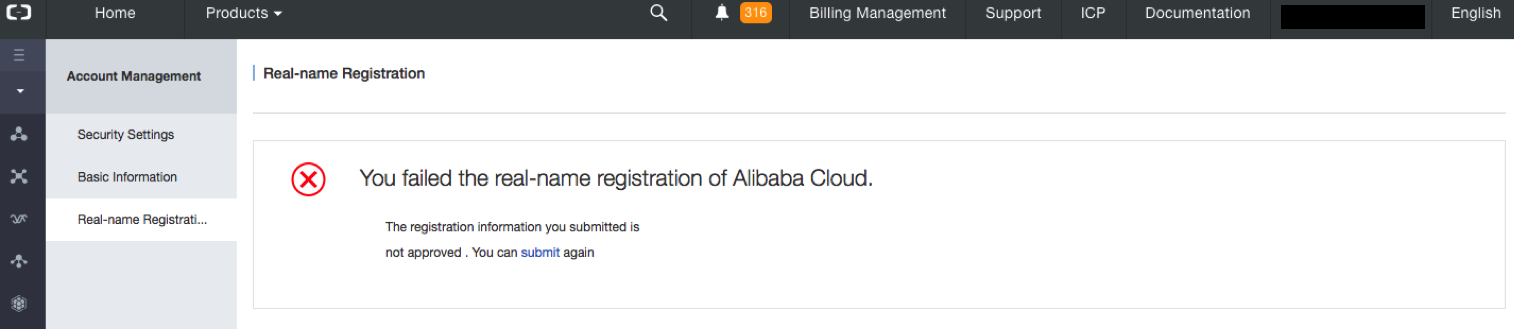A partial screenshot from a website shows two dark gray banners: one vertical on the left side and another horizontal across the top. A bold, red circle with an "X" in the center occupies the middle of the image, accompanied by the message "You failed the real name registration of Alibaba Cloud." On the left vertical banner, various clickable options are listed, including "Account Management," "Security Settings," "Basic Information," and "Real-Time Registration." The top horizontal banner has a navigation menu displaying icons and options from left to right, including "Home," "Products" with a dropdown arrow, "Billing Management," "Support," "ICP Documentation," and "English" located at the far upper right corner.